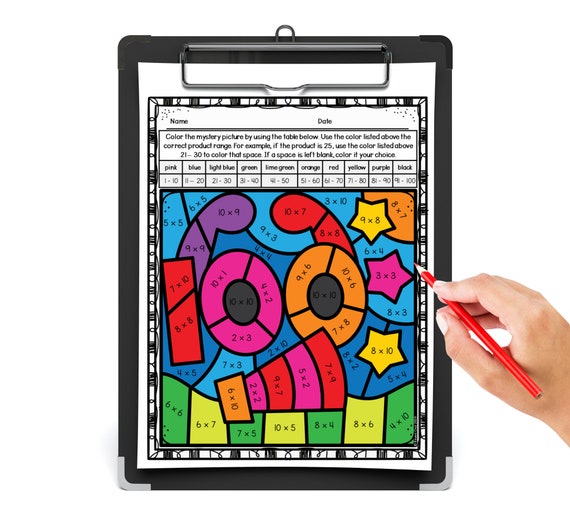The image depicts a vertically aligned rectangular black clipboard with a white sheet of paper clipped onto it by a large rectangular silver clip at the top. The paper, a coloring worksheet, has sections for a name in the upper-left corner and a date in the upper-right corner, both of which are blank. The instructions on the worksheet read, "Color the mystery picture by using the table below. Use the color listed above the correct product range. For example, if the product is 25, use the color listed above 21 to 30 to color that space. If a space is left blank, color it at your choice.” Below the instructions, there is a detailed table with color names—pink, blue, light blue, green, lime green, orange, red, yellow, purple, and black—paired with corresponding number ranges for coloring. The central image, featuring the number "100" surrounded by various rectangular and square shapes, is shaded in multiple colors according to the worksheet's guidelines. In the lower right of the image, a hand is holding a red colored pencil, poised over the paper. The overall setting is bright and clearly lit, showcasing the vivid array of colors used in the coloring activity.